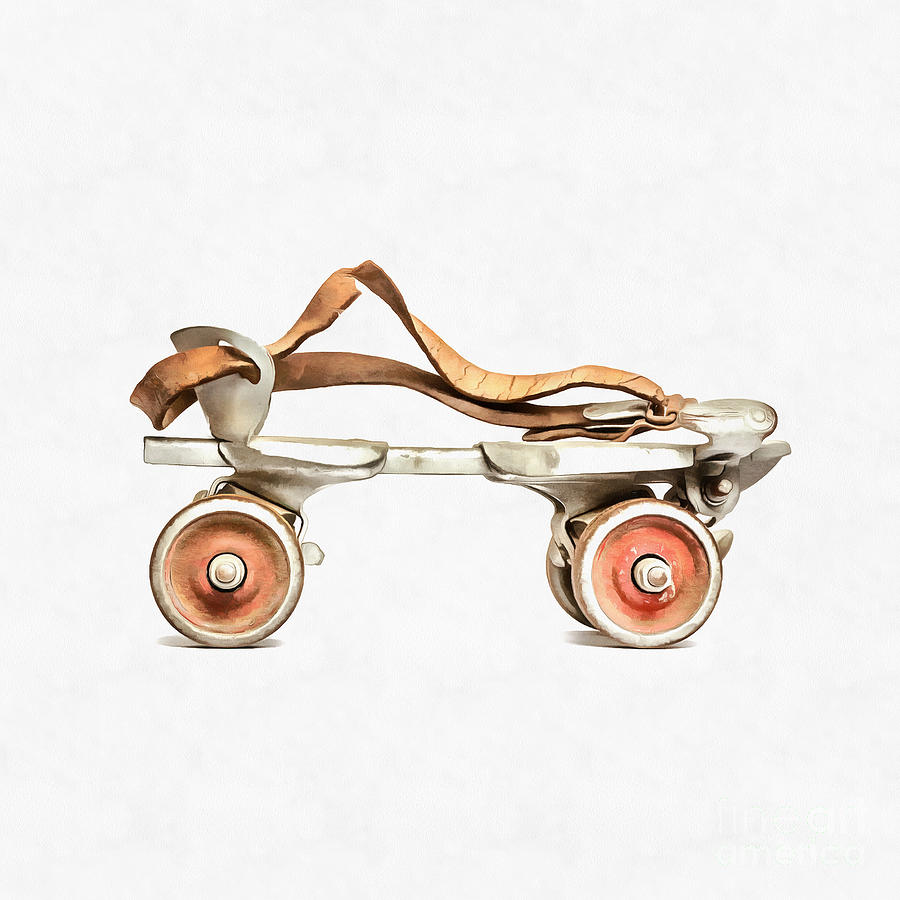The image depicts a detailed, old-fashioned roller skate in a close-up profile view, set against a plain, off-white background with some subtle patterning. This drawing or watercolor illustration showcases a unique roller skate, characterized by a combination of vintage design and distressed elements. The skate features a light brown leather strap designed to secure it to the wearer's foot, mimicking a thong sandal by positioning the strap between the big toe and the rest of the toes. The platform of the skate, where the foot would go, is primarily white with hints of silver.

The roller skate is equipped with distinctive wheels, each having a white outer rim with an orange center, and a decorative cream or pearl-like detail at the very core. Despite variations in wheel descriptions, they share a common theme of a two-toned color scheme with intricate design. The metallic frame supporting the skate is evident, with white bolts securing the hard rubber or metal wheels in place. The image also employs shading techniques, creating shadows under the wheels, and is oriented such that the viewer sees it from a side angle, revealing three wheels clearly while the fourth is partially obscured. This detailed and textured representation captures the nostalgic essence of a bygone era in roller skating.